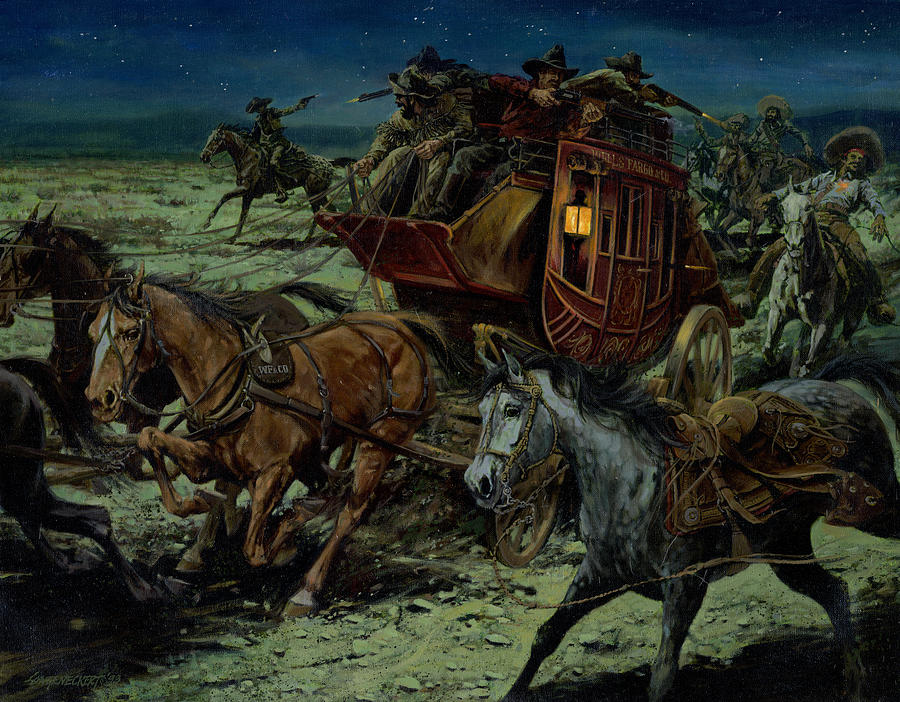An illustration evocative of the 1800s Western frontier captures the tense chaos of a stagecoach robbery under a star-studded night sky. The scene is bathed in moonlight, revealing a sandy, gravelly prairie landscape dotted with sparse shrubs and shadowed silhouettes of distant mountains. Central to the image is a Wells Fargo stagecoach, hurtling diagonally from right to left, pulled by three horses in full gallop. The driver, reins in hand, leans forward with a determined expression as two other men atop the stagecoach fire their rifles. Surrounding them are four to five bandits on horseback, engaged in a fierce gunfight, each donning cowboy hats and bullet sashes. Amid the chaos, a grey Appaloosa horse without a rider bolts across the bottom right corner, suggesting a prior skirmish or casualty. The atmosphere is charged, the ground bearing indents from the frantic pace of the horses, as the stagecoach and its defenders fight desperately against their relentless attackers.